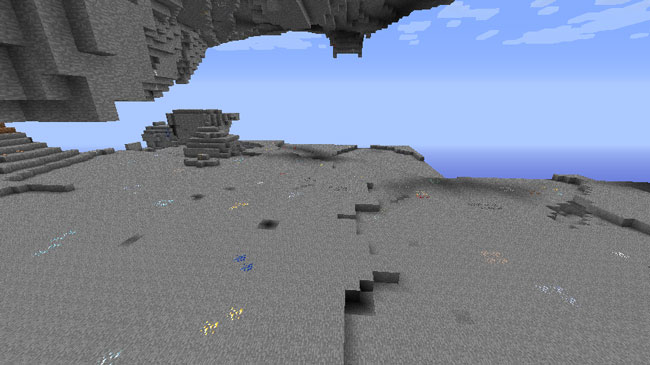The image showcases a striking rock or cement structure, resembling an architectural marvel suspended high in the sky. The platform, which appears to be cement-covered, features a prominent rock overhang on the top, creating the illusion of a roof. The structure begins narrow on the left side and gradually widens to the right, unveiling an expansive view of a blue sky streaked with wispy clouds.

From the center left, a series of six to eight cement steps descend to a gray stone or cement platform that dominates the entire lower half of the image. The platform exhibits subtle variations in elevation, being higher on the left and gradually sloping down to the right, adding depth and dimension to the scene.

The upper left corner of the image reveals a blend of cement and natural rock textures, characterized by sharp geometric angles that give way to a more organic, rugged appearance towards the center top. Shadows and intricate details enhance the contrast and texture, making the structure appear both man-made and naturally integrated into its sky-high setting. The overall composition captures the rugged elegance of the design, accentuated by the interplay of light and shadow, and the vast, ethereal backdrop of the sky.